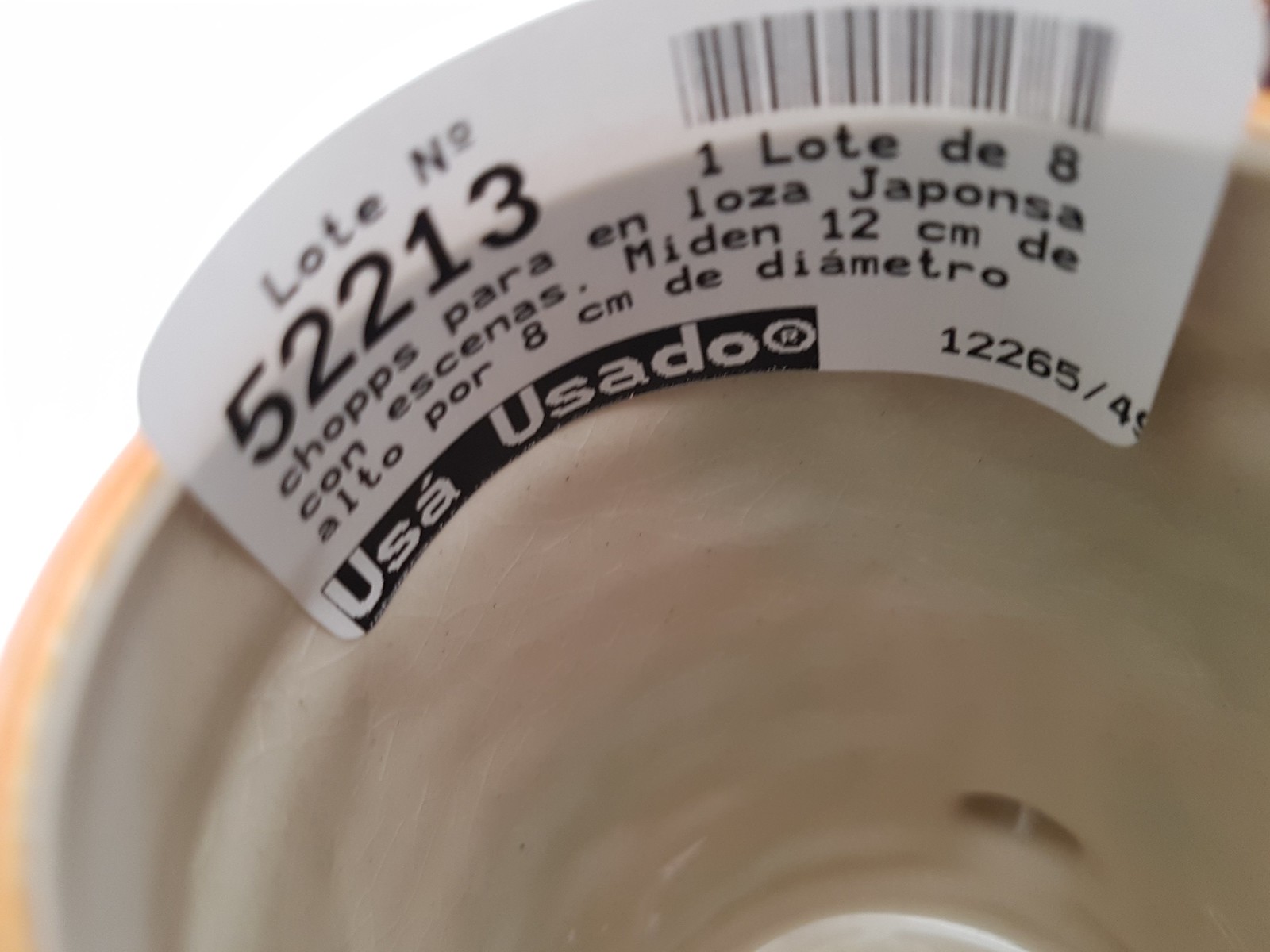The photograph captures a close-up of a white paper sticker label adhered to a pottery item, likely a vase or vessel, showcasing its glazed surface adorned with fine cracks running vertically along its tubular form. The backdrop is a pristine white, providing a clear contrast to the intricate details of the pottery. Prominently printed on the label is a black UPC barcode with the number "52213" adjacent to it, adding a touch of modernity to the traditional craftsmanship of the pottery.